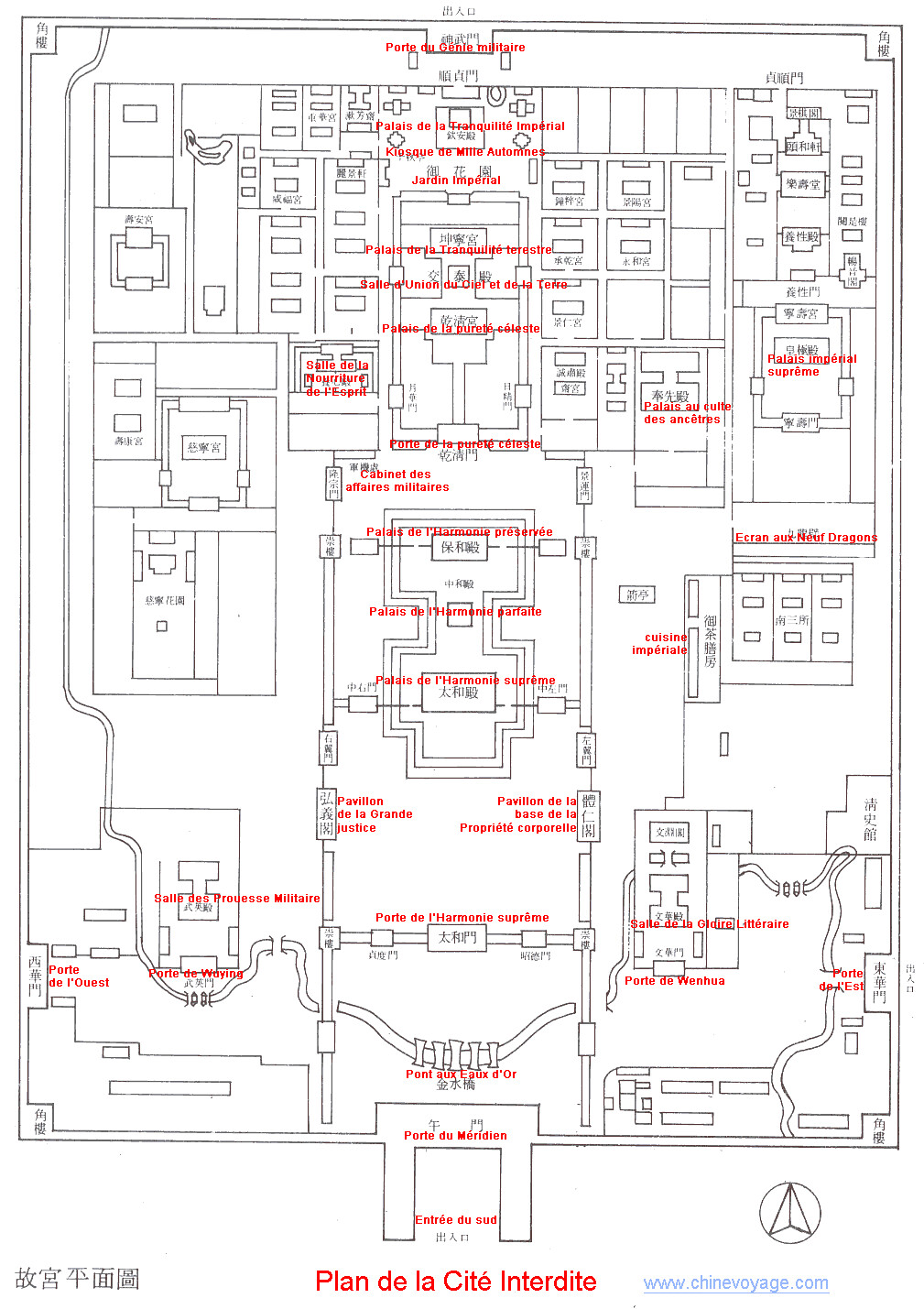This image showcases a detailed black-and-white architectural blueprint of a building floor plan, intricately hand-drawn and annotated. Dominating the blueprint is the title "Plan de la Cité Interdite" in red text, indicating a possibly French colonial influence. Noteworthy are the numerous labels, approximately twenty in total, and an arrow on the lower right side suggesting directionality, though it is not marked with an 'N'. The plan features an entrance leading to multiple smaller subdivided rooms and hallways, including some areas likely allocated for engineering purposes.

The blueprint includes other notable markings in red and a mixture of foreign text—specifically Asian characters, possibly Chinese or Japanese, and smaller print that's largely unreadable due to its size. The presence of Asian writing hints at an Indo-Chinese connection. At the bottom, the legend or identifying mark includes a link to Chinesevoyage.com, alluding to its origin or the context of its use. This meticulous floor plan encapsulates a structured and comprehensive layout, indicative of a significant architectural endeavor.